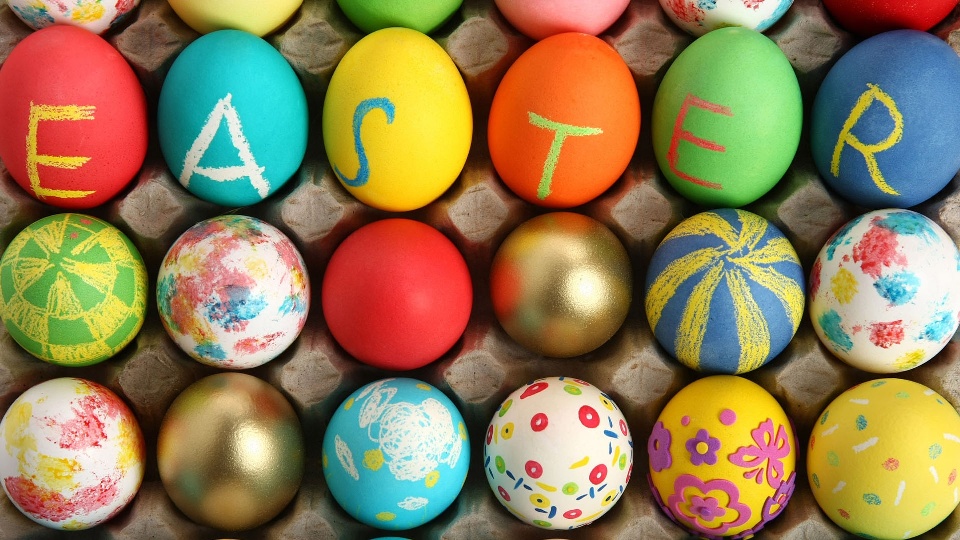This image captures a top-down view of a typical gray styrofoam egg carton filled with brightly decorated Easter eggs. The carton has four rows and seven columns. The second row from the top features eggs that spell out "EASTER," with one letter per egg: a red egg with a yellow 'E', a turquoise egg with a white 'A', a yellow egg with a turquoise 'S', an orange egg with a lime green 'T', a light green egg with a pink 'E', and a purplish-blue egg with a yellow 'R'. These eggs are solid-colored. Below this row, the eggs exhibit a variety of decorations, including metallic hues, printed patterns, dye effects, foam stickers, and hand-drawn chalk designs creating checker patterns and geometric shapes. Each egg is uniquely adorned, contributing to a vibrant and festive visual display.